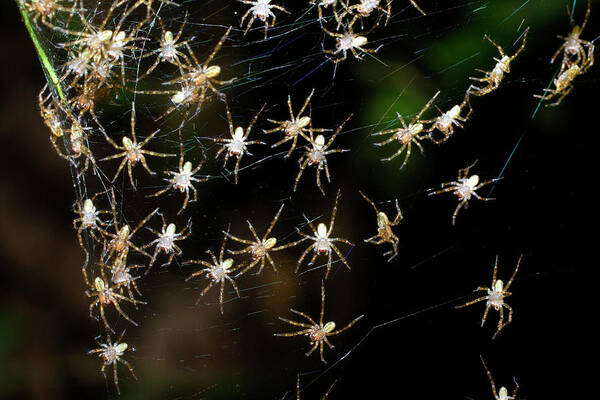This close-up photograph showcases a dense web populated by numerous small spiders, estimated to be around 20 to 30 in number. Primarily concentrated in the left center portion of the image, these spiders exhibit light-colored bodies with segmented legs, varying in shades from white to beige and brown. Their abdomens are notably lighter. The spiders are scattered throughout the intricate web, with notable clusters: a trio is situated at the top center, with another spider nearby, and similar groupings of spiders appear towards the top right and center-right of the frame. A soft, blurred green backdrop with hints of dark brown adds depth to the composition, suggesting foliage in the background. The overall effect is reminiscent of fireflies due to the spiders’ light-colored bodies glowing against the web’s darker threads. This image probably captures a group of young spiders congregating before they disperse, hinting at the unseen presence of their mother nearby.